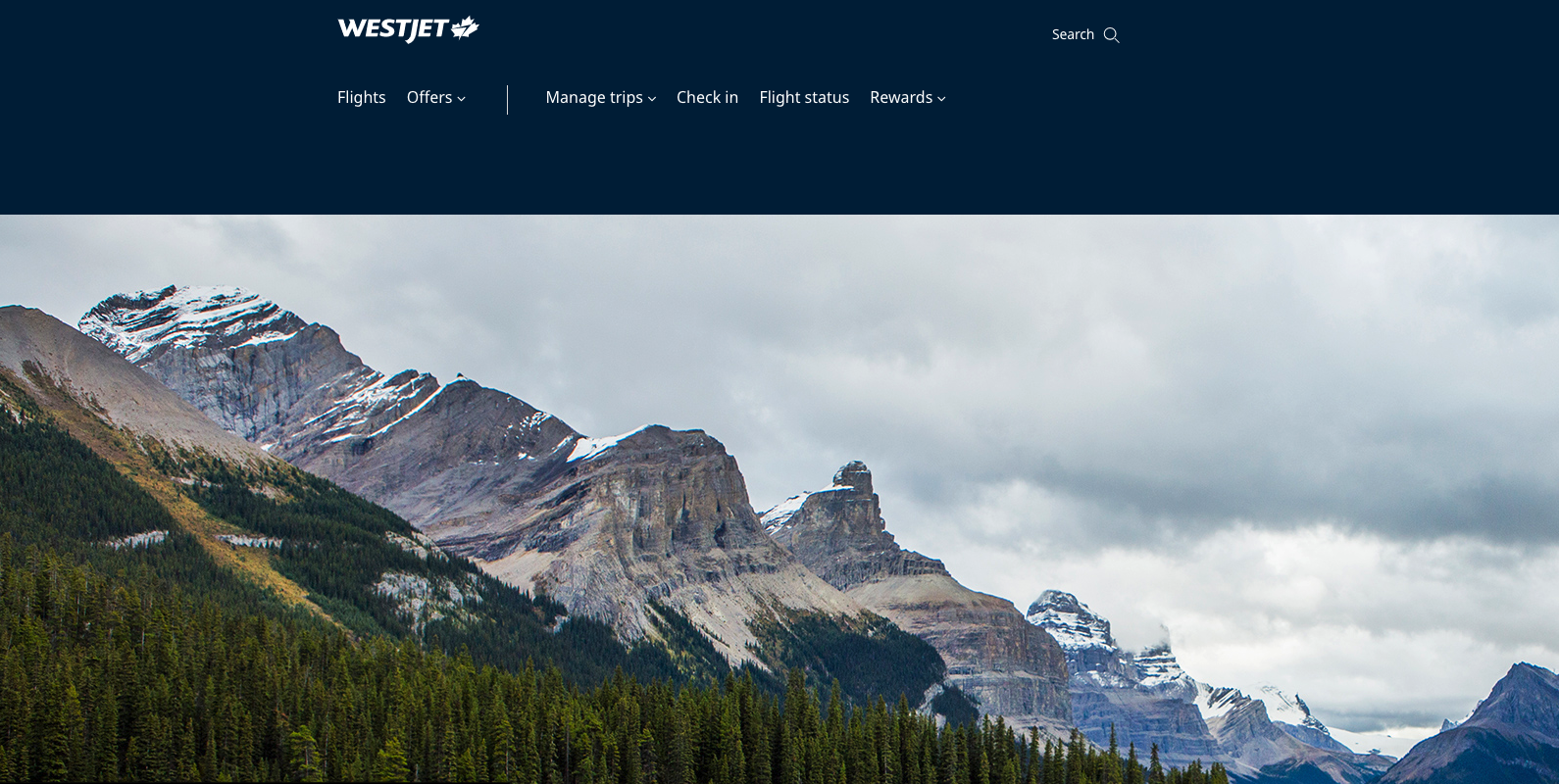In this particular image, we see the homepage of the WestJet website. The company's name, "WESTJET," is prominently displayed in all capital letters with their logo beside it. On the far right of the header, there's a search icon accompanied by the word "Search" and a search box. Below this main header, there is a menu bar featuring several categories: "Flights," "Offers," followed by a small dividing line. Post the divider, the menu continues with "Manage Trips," "Check-in," "Flight Status," and "Rewards." This entire header section features a sleek black background.

Directly below the header, the viewer is greeted by a breathtaking image of a mountainous landscape. These mountains are topped with patches of snow and are light brown with some darker areas. A uniformly spread band of trees spans from the left to the right side of the screen. Above the mountains, the sky is filled with ominous, dark clouds with hints of white, adding depth and contrast to the scenery. The menu items under the "WestJet" header are rendered in small but legible text.